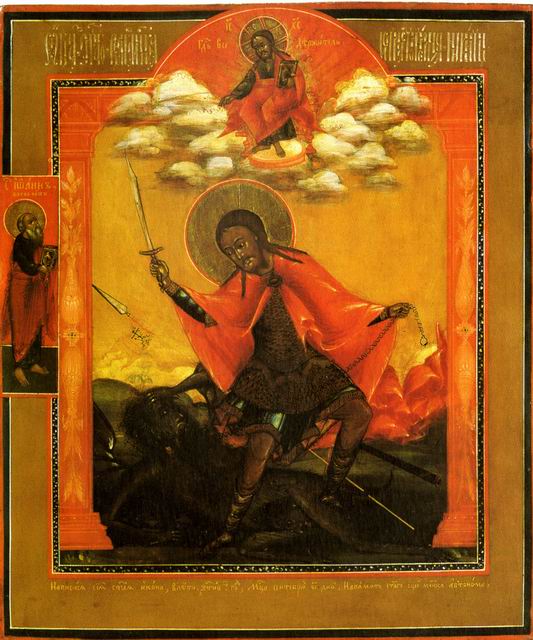This image is a highly detailed painting with religious iconography featuring saint-like figures adorned with halos. Centrally, a dark-skinned warrior akin to a samurai, with tightly braided dark brown hair and dark attire, stands prominently. He wears a shiny, orange-red cloak that could be compared to a slick, plasticky material. A rounded hat obscures part of his face, and he holds a raised sword while his other hand clutches a chain. Underneath his cloak, he seems to be dressed in dark armor or a military uniform, complete with dark black boots.

Standing on what appears to be a dark road marked by a white line, suggesting an old street, the central figure is framed by a complex border. This border consists of multiple narrow bandings of black, gold, red, white, and black again—a combination giving depth and prominence to the figure.

Above the central warrior, another smaller figure, possibly a saint, floats on golden clouds. This figure, appearing ethereal with a halo, also dons a red cloak and holds a book. To the left, another haloed figure with black sleeves and a red skirt also clutches a book, contributing to the religious theme.

Adding to the sanctified aura, finely written yellow text over light gold decorates the bottom, while more text in another language appears at the top. These elements, along with the black frame around the gold border, encapsulate the mystical and historic essence of the painting. 

Overall, the intricate details, religious symbolism, and layered framing make this painting a rich and evocative piece of art.